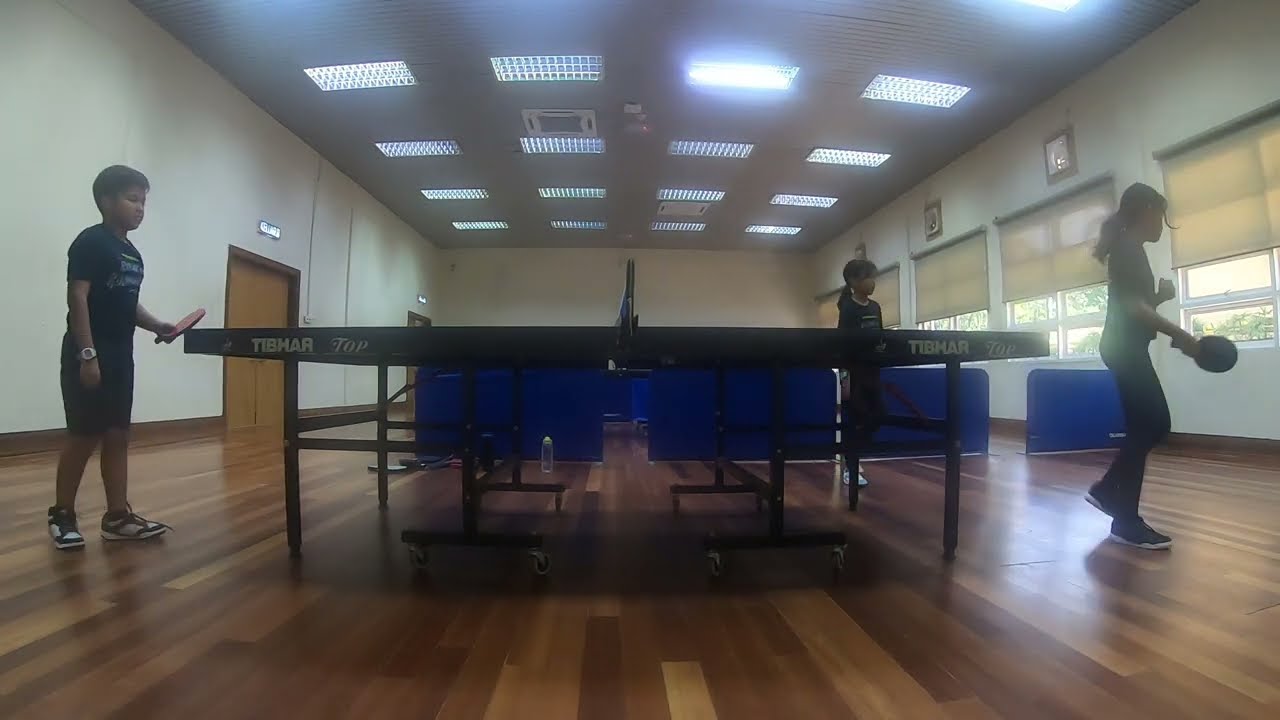In a bright, well-lit room with tile ceilings and wooden floors, three young children are engrossed in a game of ping-pong at the center. The boy, wearing a blue shirt and black shorts, stands at the left end of the ping-pong table, his paddle resting on the table with a watch on his wrist. Opposite him, a girl with a ponytail, likely of Asian descent, stands poised with her paddle, while another girl, also appearing to be of Asian descent and dressed in dark clothing, walks away, perhaps to retrieve a ball. This girl, on the right side, holds a ping-pong paddle, indicating her participation in the game. The ping-pong table, sporting the logo "Tib Mar Top," stands on wheels and has a water bottle beneath it. Behind it, blue cloth barriers section off the area. The room's walls are crisp white, with two wooden doors set further back on the left and four windows with shades halfway drawn down on the right. This scene likely unfolds in a recreation center or gym, suggested by the setup and the focus on play and activity.